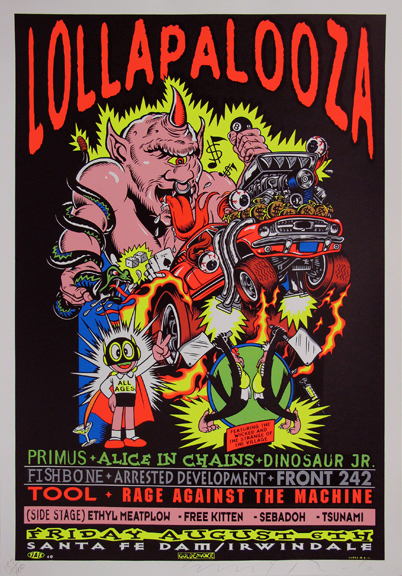This is a highly colorful and vibrant concert poster for Lollapalooza, featuring an eye-catching design in vivid neon hues of orange, yellow, green, and pink. Styled in the cartoonish, psychedelic art reminiscent of R. Crumb and 1960s counterculture, the poster prominently displays a muscular and sinister figure resembling a genie or demon. This character is a cyclops with a single eye, a red horn protruding from its forehead, a forked tongue, and pointed ears. A snake coils around his arm as he grips a magic 8-ball gear shift attached to a diminutive hot rod filled with coins and eyeballs. 

Below the central figure is a small, caped superhero-like character, adding to the eclectic and whimsical nature of the artwork. Additional cartoonish figures can be seen, reminiscent of Mad Magazine illustrations, engaging in playful antics.

At the top of the poster, "Lollapalooza" is emblazoned in red letters, beneath which the lineup of performing bands is listed: Primus, Alice in Chains, Dinosaur Jr., Fishbone, Arrested Development, Front 242, Tool, and Rage Against the Machine. Side Stage performances by Ethel Meat Plow, Free Kitten, Cebado, and Tsunami are also included. The event is scheduled for Friday, August 6th at the Santa Fe Dam in Irwindale. The saturated colors and dynamic imagery capture the energetic and rebellious spirit of the Lollapalooza festival.